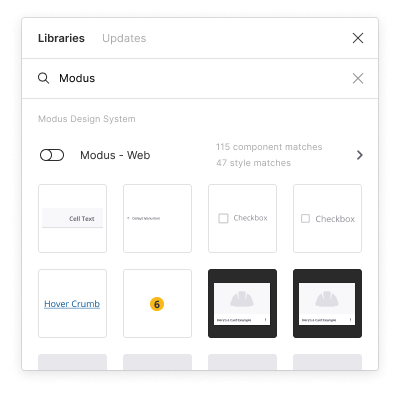This screenshot captures a section of a software or web application, focusing on a search result page for "Modus" within the "Libraries" section. The image has been cropped, removing some contextual information. The background is predominantly white. At the top, there's a search bar with "Modus" entered as the search term. The highlighted area provides information about the search results, stating "115 component matches, 47 style matches."

Displayed prominently are search results related to "Modus design systems." The results are organized into square boxes, each representing different web design elements. Currently, 8 of these elements are visible. They include varied items like a checkbox, a hyperlink hover crumb, distinct text styles, and a number 6 encased in a yellow circle. The design elements showcased reflect the diversity of the components and styles found within the "Modus" search results, indicating a broad array of tools and options available in the design system.